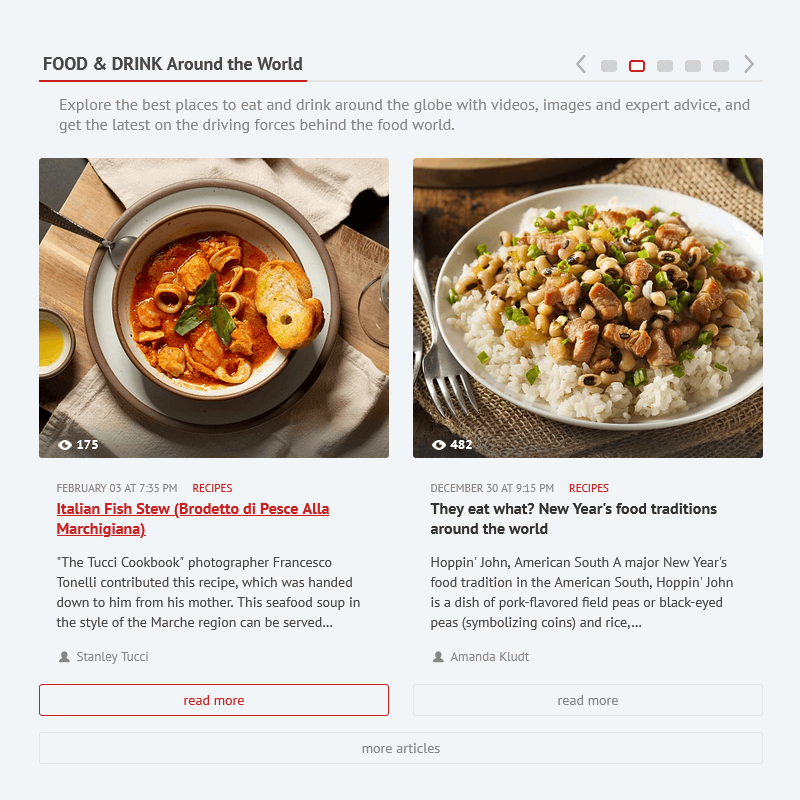The image is a screenshot of a website titled "FOOD AND DRINK AROUND THE WORLD" in bold, capitalized black text underlined with a red line. On the right side of the page, there are five numbered gray boxes, with the second box outlined in red. 

The highlighted section reads: "Explore the best places to eat and drink around the globe with videos, images, and expert advice. Get the latest on the driving forces behind the food world." Below this text is an image depicting a bowl of soup, which appears to be a fish stew, garnished with a green leaf and accompanied by a piece of toasted bread. The bowl, resting on a plate that matches its design, has a spoon placed on the side. A yellow sauce is visible next to the bowl, which is set on a cloth napkin.

Underneath the image, the caption reads: "Italian Fish Stew - Burrito di Pesce alla Margiana. This recipe, contributed by 'The Tushy Cookbook' photographer Francisco Tonell, was handed down to him from his mother. The seafood soup in the style of the Marsha region can be..." The caption ends with a "Read More" button in a red box.

Another image is numbered 482, depicting rice topped with chicken and vegetables, showcasing visible greens. The accompanying caption talks about New Year's food traditions around the world and specifically mentions "Hoppin' John - American South. A major New Year's tradition in the American South, Hoppin' John is a dish of pork-flavored field peas or black-eyed peas symbolizing coins and rice."